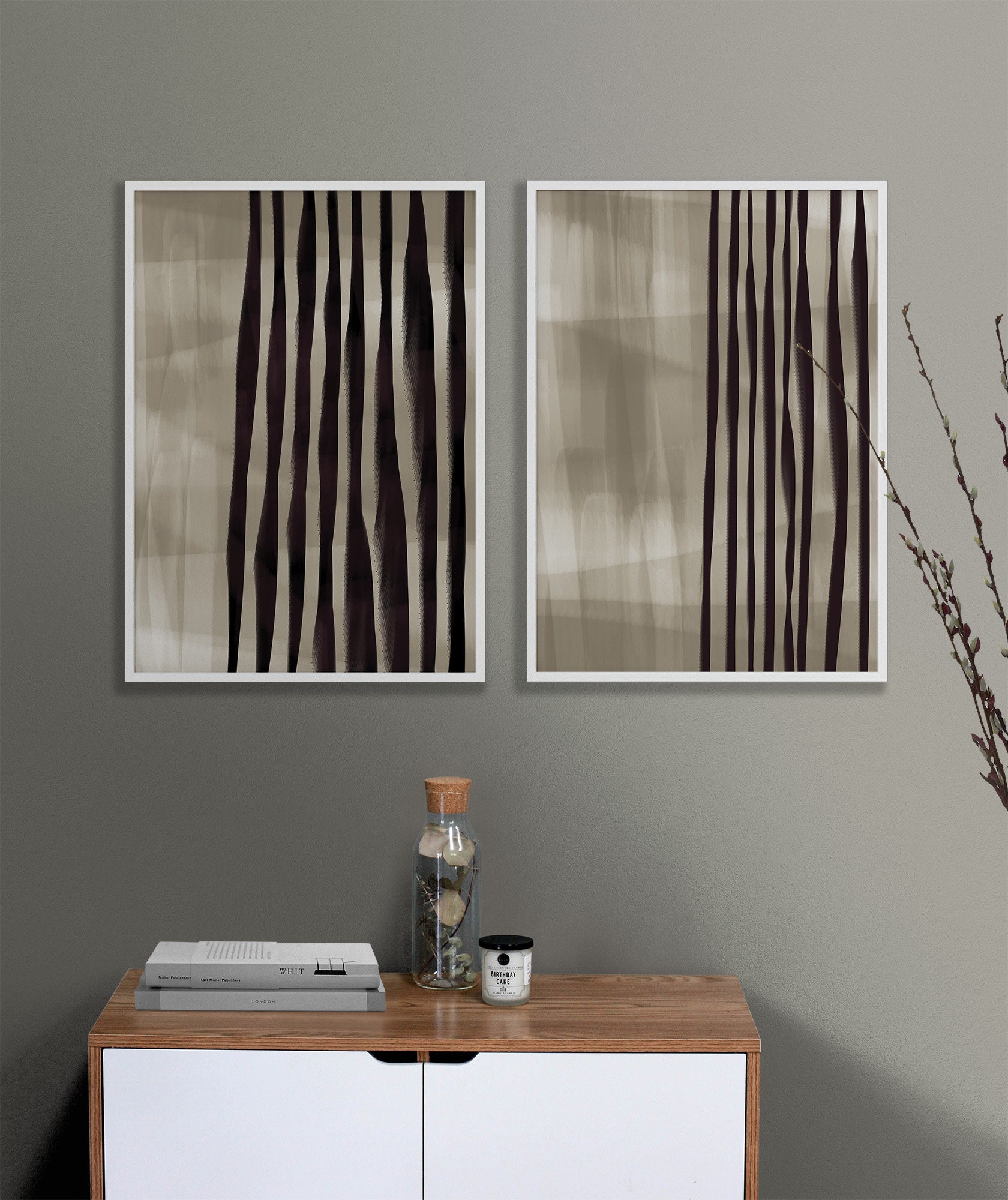The photograph depicts a professionally taken, vertically oriented scene set against a gray wall. Centrally, a wooden cabinet with white doors serves as a focal point. Atop the cabinet lies a neatly arranged still life: two coffee table books, a glass container with a cork top holding decorative accents, and a white candle with a black lid, featuring some indistinct text. To the right, the tips of a plant, possibly cattails or pussy willows, peek into the frame, adding a natural touch to the composition.

Dominating the visual narrative are two vertically oriented, modern art paintings hung side by side on the wall. Encased in white frames, these artworks feature a beige-to-gray blurred background accentuated by black vertical stripes occupying most of the right side, with subtle triangular shapes and brush strokes enhancing their abstract quality. Together, these elements create a refined, stylish scene, suggestive of a carefully curated living room space.